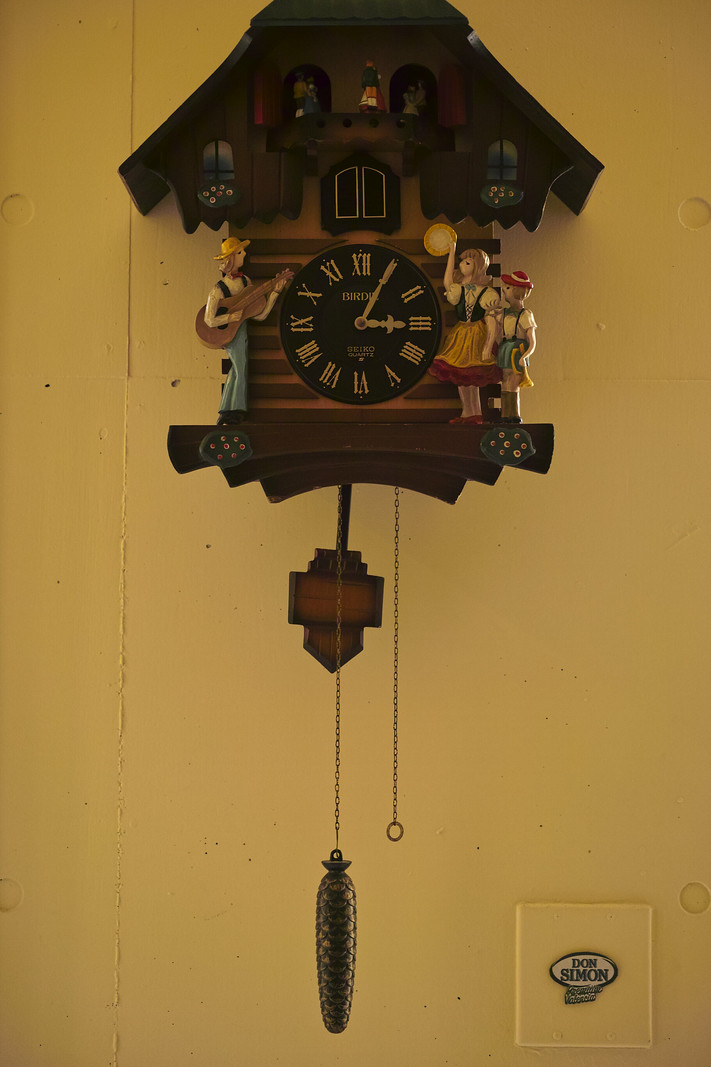This photograph captures an elaborately detailed cuckoo clock, adorned with intricate features. The top of the clock is designed to resemble a forest, painted in an olive green hue, and showcases a group of dancing figurines standing on a balcony. Flanking them are two windows framed by flowering bushes. Just below the balcony are dark shutters embellished with yellow trim. 

The clock face, set in a very dark green backdrop, features pale yellow Roman numerals and matching clock hands. On either side of the clock face stand human figures; one wears a yellow hat and is playing a guitar, while another, a woman in a skirt of yellow and burgundy, holds a yellow circular object. Beside her is another figure adorned with a red and white hat, all standing on a wooden platform decorated with flowering bushes. 

Below this platform swings a pendulum in hues of gold and brown. Additionally, there hangs a metal object with black and gold coloring, alongside a dangling chain. Attached to the wall is a small yellow square object inscribed with the name "Don Simon".